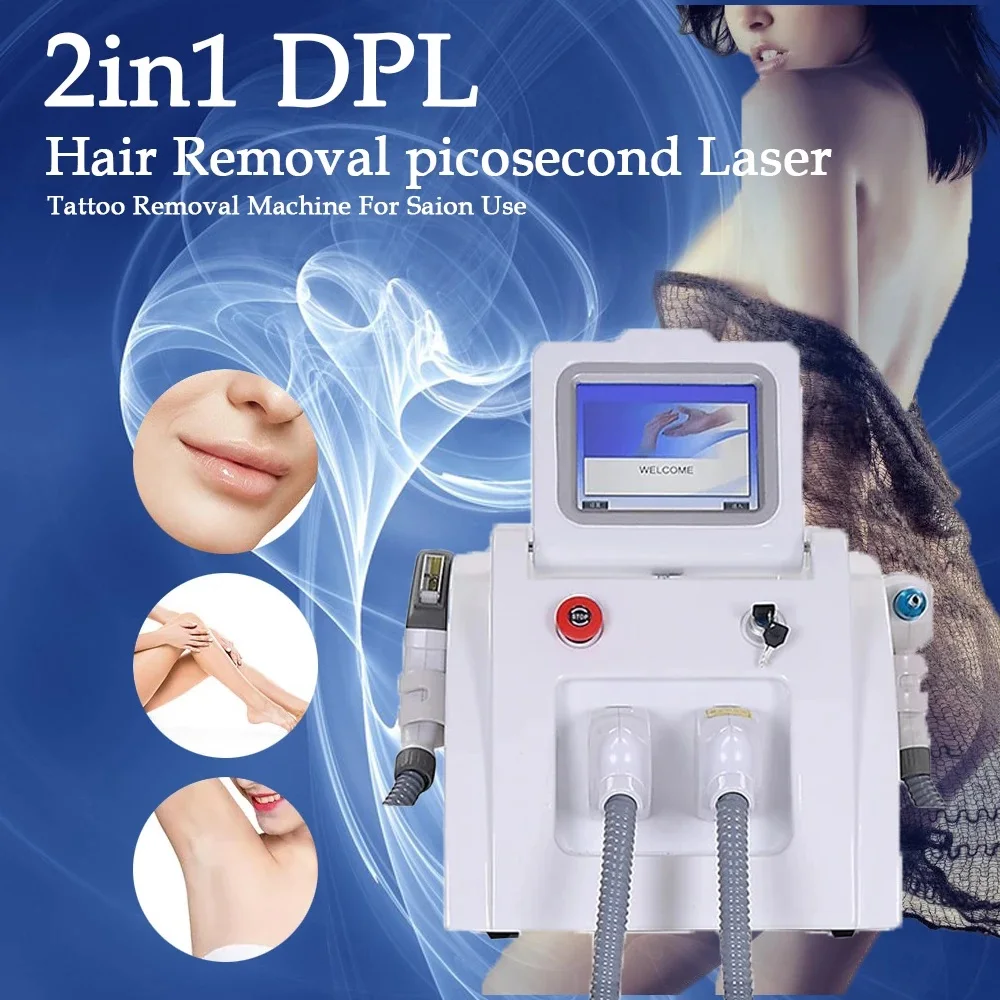This detailed advertisement poster features a 2-in-1 DPL hair removal and picosecond laser tattoo removal machine for salon use. The background is a rich blue, with bold white lettering at the top-left corner detailing the product's name and functionality. Central to the composition is the sleek, white-and-gray laser device, resembling a miniature robot with tubes and knobs extending from it. To its left are three circular images showcasing areas commonly treated: a woman's upper lip, her legs, and her underarm. On the right side stands a scantily clad woman, facing left, wearing sheer fabric that reveals her smooth, clear skin, suggesting the effectiveness of the machine. Her shoulder-length dark hair partially conceals her eyes, highlighting her mouth and nose. This image collectively conveys the device’s capabilities in providing smooth, hair-free, and tattoo-free skin.